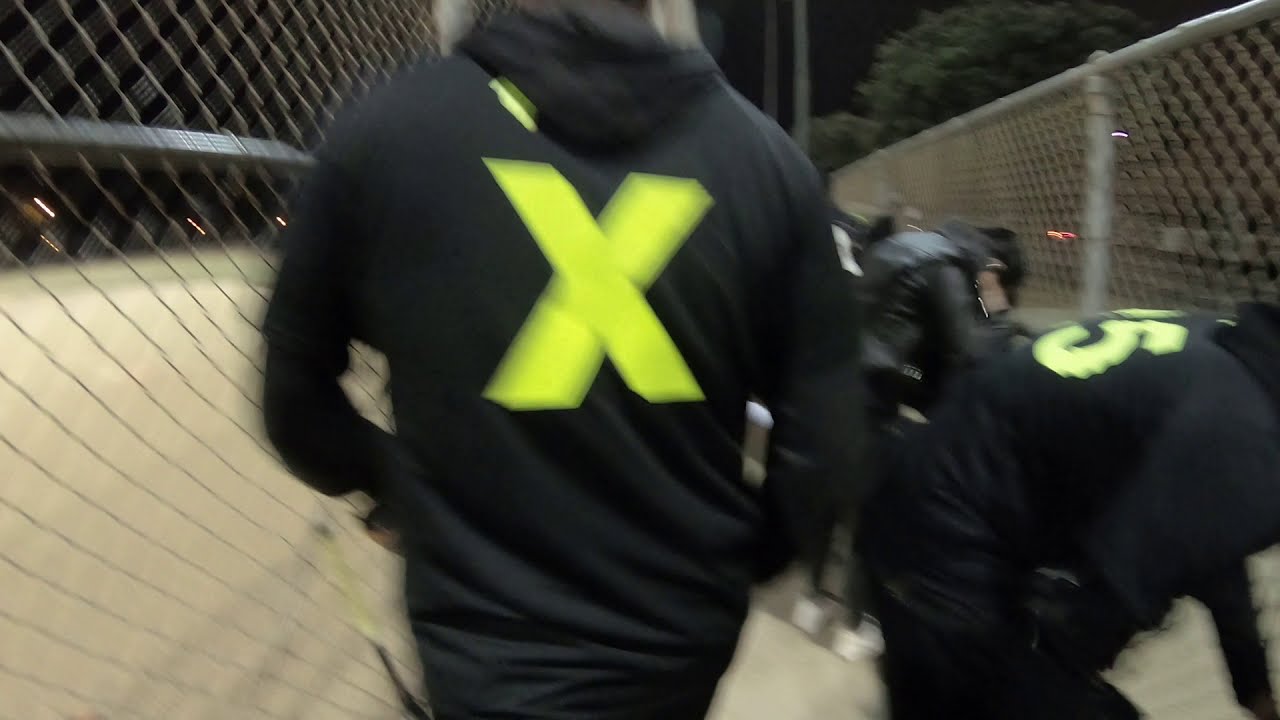In the image, amid a blur of motion, several men stand within a narrow outdoor passage flanked by metal fences on both sides. Dominating the foreground, a man in a black hoodie emblazoned with a yellow 'X' on his back faces away from the camera. To his right, another man, slightly slouched towards the fence, wears a similar black outfit with a yellow '5' visible on his back. This second man is accompanied by two additional individuals, all attired in black and white ensembles. The men, possibly SWAT members or security personnel, seem to be coordinating an operation, their movements captured in a candid, dynamic moment that leaves their faces obscured and the exact nature of their activity open to interpretation.